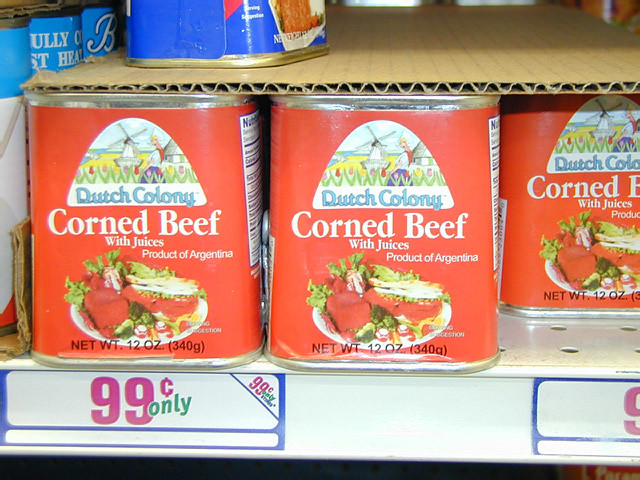A close-up photograph taken in a grocery store, showcasing a shelf stocked with corned beef. Three neatly arranged rows of the product are visible, each featuring a red, rectangular container similar in shape to a soup can. The label on the cans reads "Dutch Colony Corned Beef," indicating that it is a product of Argentina and weighs 12 ounces. Priced at 99 cents each, according to the small shelf tag, the corned beef cans capture attention. However, one of the cans is slightly pushed back, breaking the otherwise uniform alignment. Above the rows of corned beef, a piece of cardboard supports a single blue can, adding a contrasting detail to the display.